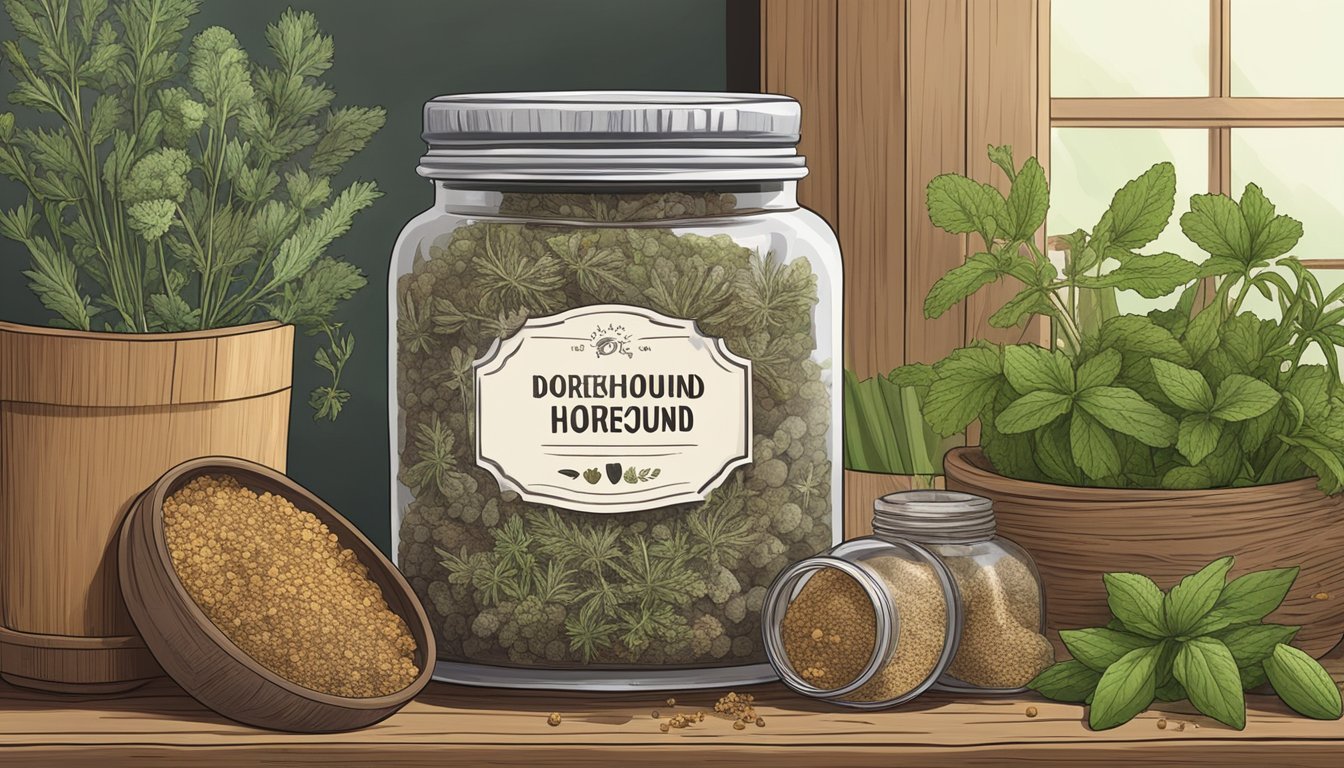This colorized illustration depicts a detailed scene of a wooden shelf laden with various herbs and containers, set against a backdrop of matching woodwork framing a windowpane, with a dark gray wall in the background. Dominating the foreground is a large glass jar with a silver metal lid, labeled "whorehound" in multiple languages, and filled with dried green herbs that resemble marijuana buds. To the left of the jar, a tan flower pot brims with lush green plants, while to the right, a wooden container holds tall, leafy stalks emerging prominently. Additional details include a brown bowl leaning against the wooden pot, filled with some type of brown material or seeds, and nearby, a couple of smaller jars also filled with similar seeds, one of which is tipped over with a silver lid beside it. The subdued color palette and intricate detailing allow us to appreciate the texture of the wooden surfaces, the granules of the spices, and the shape of the leaves.